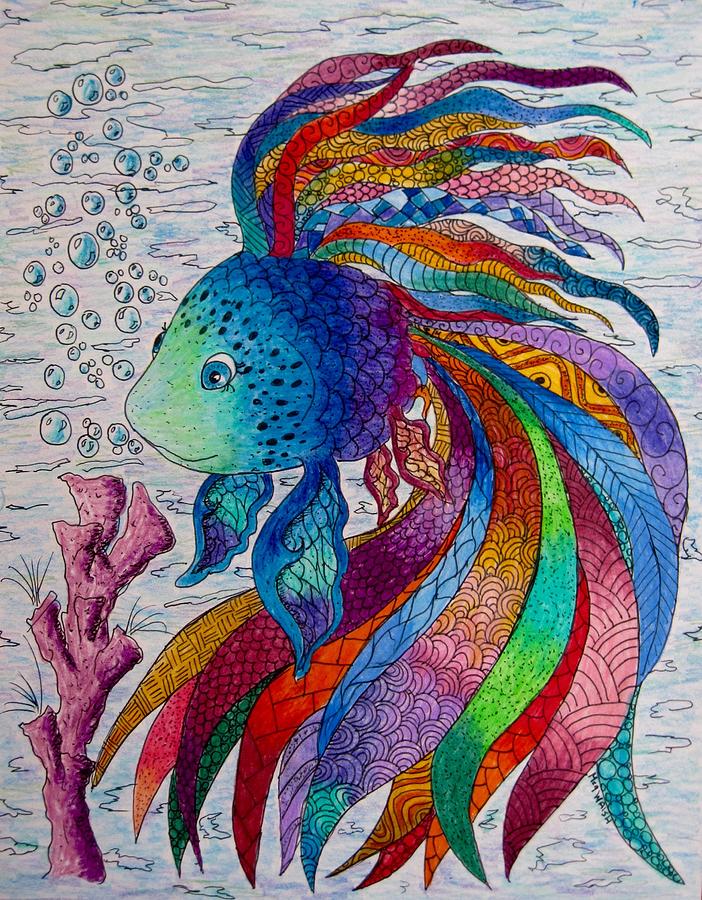This detailed and vibrant illustration depicts a hand-drawn and intricately colored fish, resembling a fusion of fantasy and marine life. The fish, with a body shape akin to a goldfish, showcases an array of rich hues, transitioning from light teal at its head, which has a humanlike face with blue eyes and black pupils, to deep blue and purple towards its tail. The artist's signature, though difficult to decipher, appears to be "Walsh." The fish's fins and tail are adorned with an elaborate collection of ribbon-like streamers in a spectrum of colors including purple, yellow, pink, green, red, and blue, each displaying unique patterns without a set arrangement. These streamers extend gracefully, almost filling the entire right side of the canvas and trailing towards the bottom, giving the impression of movement. The scene is set underwater, with the fish surrounded by small, air bubbles rising upwards. Adjacent to the fish, a vibrant purple coral reef stretches upward, adding to the illustration's sense of depth and aquatic atmosphere. The fish's gaze is directed to the left, giving a serene yet mesmerizing focal point in the colorful seascape.